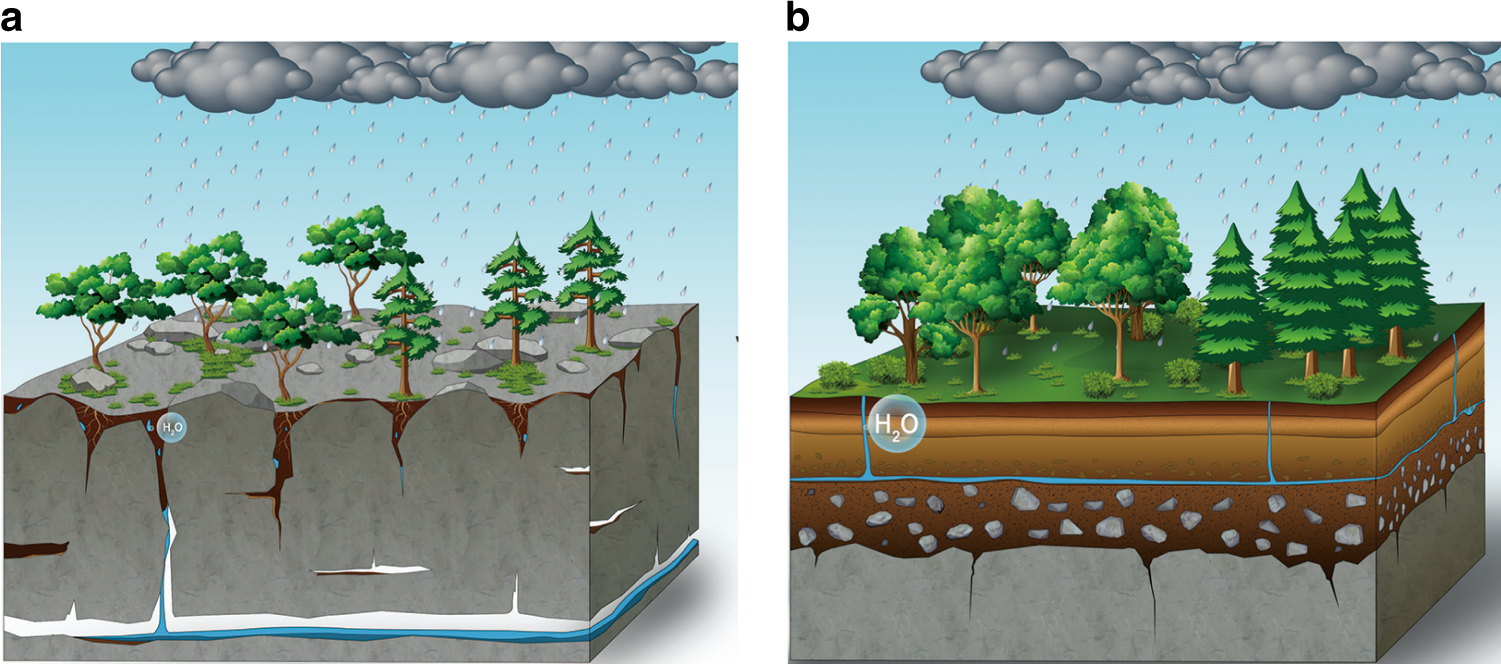The image features two square, animated pictures labeled A and B, positioned side by side with A on the left and B on the right. Both pictures illustrate land structures shaped like short cubes with raindrops falling from gray clouds, highlighting differences in soil, rock, and vegetation.

In image A, the cube-shaped land structure displays a predominantly grey, rocky top surface with sparse, less full trees and patches of green grass. The front face of the cube reveals brown soil beneath the trees, with white lines indicating water seepage that pools under the rock and then runs off via a small blue line. A bubble with "H2O" is placed beside this structure to denote the presence of water.

Contrastingly, image B shows a more fertile and vibrant landscape. This left-section cube's top surface is greener, populated by fuller and healthier trees. Below the surface, the front face of the cube is mostly brown soil, traversed by blue lines indicating water pooling and remaining within the soil layer, rather than running off. More extensive soil integration with rocks is visible at the bottom edge of the cube, indicating a richer, more porous ground.

Together, these images compare two different ecosystem states, highlighting contrast in soil composition, water behavior, and tree health despite similar external conditions.